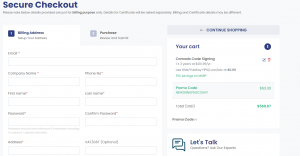The image appears to be a screenshot of a multi-step e-commerce checkout process, containing several prominent headings and sections, although portions of the text are blurry and difficult to decipher.

At the top, on a background that is very light gray or almost off-white, the heading "Secure Checkout" is clearly visible in blue on the upper left-hand side. Beneath this heading, there are several lines of black text that are not legible due to the blurriness.

To the right, there is what appears to be different tabs associated with the checkout process. The first tab, which appears to have a white background, includes a blue box labeled with the number "1." Within this section, the text "Building Address" could possibly be in blue, followed by several input fields for data entry. Above these input fields, there are likely instructions or labels, although the words are not clear. Red asterisks next to each input field indicate that the information is required.

Next to this section, there is another box, possibly gray in color, labeled either "2" or "3" with black text below it that reads "Purchases." Further black text is present underneath this heading, although it is too blurry to read.

Further along, in a blue heading, there is a section labeled "Your Cart," accompanied by a blue circle with the number "1" inside it. Below "Your Cart," there are several lines of text in black and green, but the content is not legible. 

At the bottom of the image, the phrase "Let's Talk" is prominently displayed in blue.

Overall, the layout is designed to guide the user through a secure checkout process, with clear headings and mandatory fields, despite the blurriness obstructing full readability.